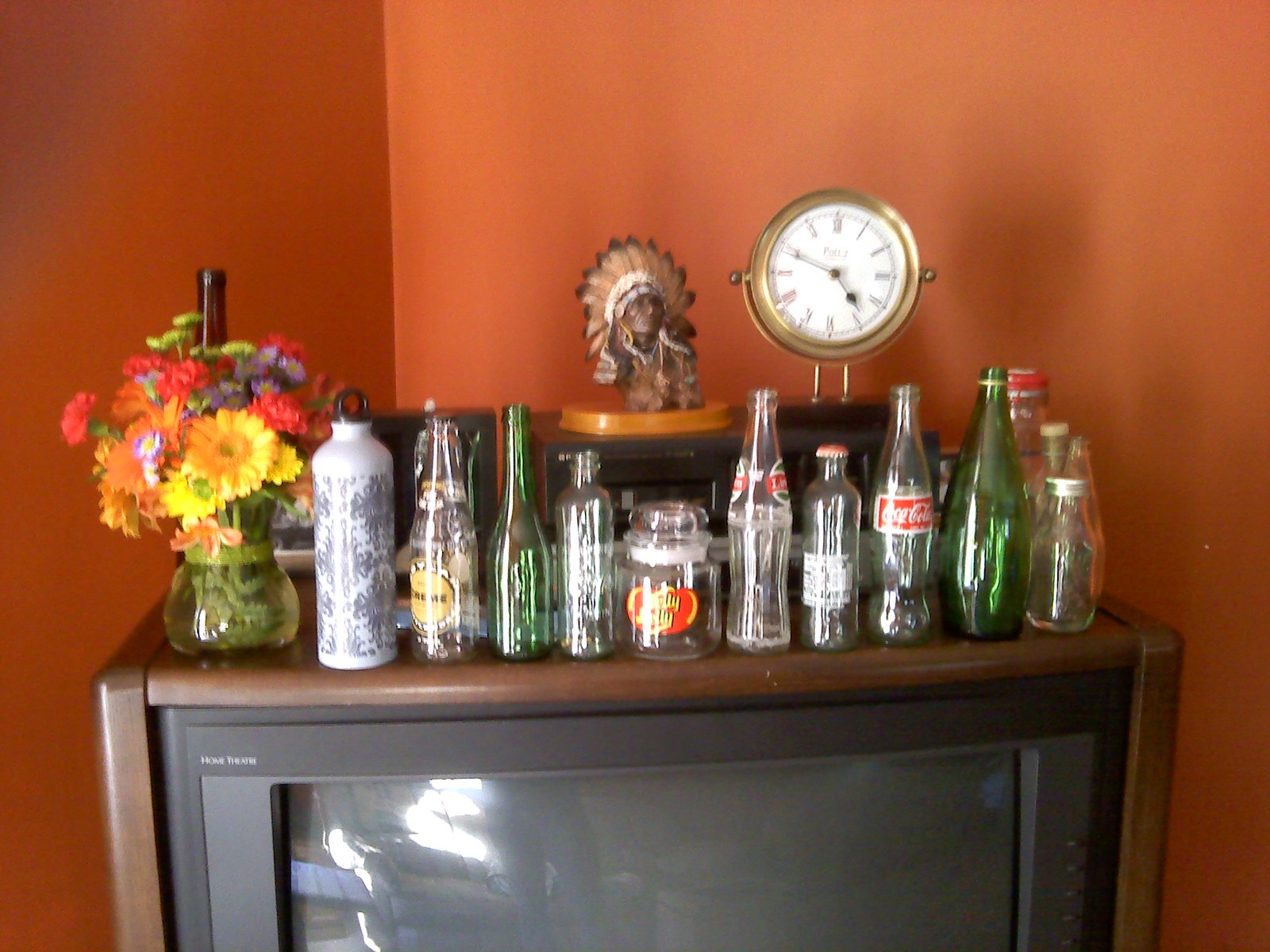In a cozy corner adorned with burnt orange walls, an old-fashioned CRT Television takes center stage, encased in a wooden frame. This black TV, switched off, features a 'Home Theater' emblem on its top left. Multiple intriguing items adorn its surface: on the far left, a clear glass vase brims with vibrant flowers. Next to it, a mix of vintage beer and soda bottles stand in a row, including a recognizable Coca-Cola bottle and a Jelly Belly jar. Among these treasures, a distinct white glass bottle also stands out. Towards the right, a small clock with Roman numerals stands guard, alongside a sculpted bust of a Native American man, replete with feathers. The reflective black screen of the TV mirrors this delightful assortment of nostalgia, creating a captivating blend of old-world charm and homely warmth.